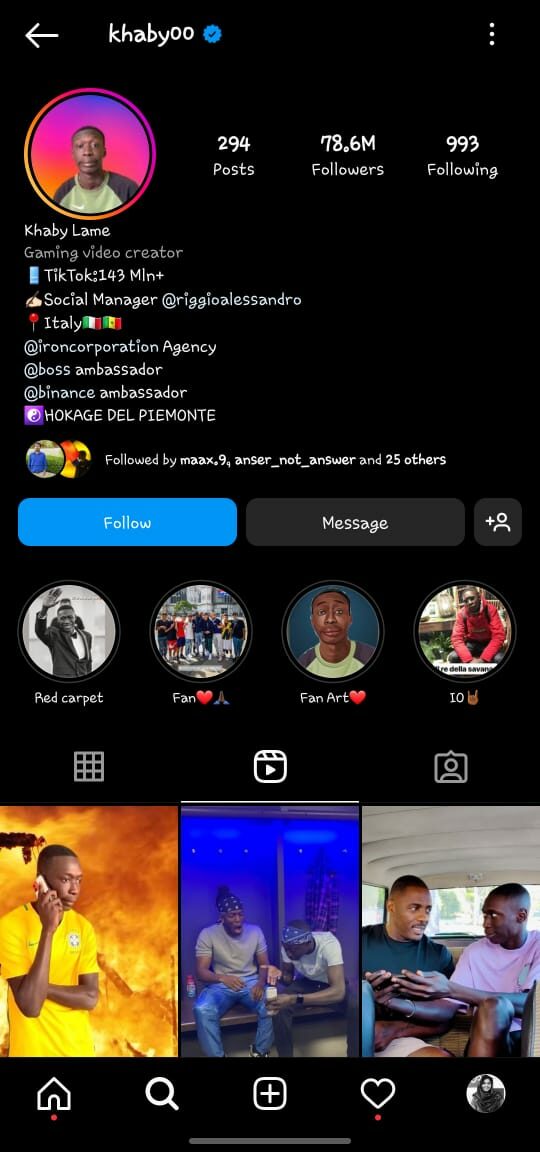Screenshot of Khaby Lame's Twitter Profile - The screen is predominantly black, featuring the Twitter interface of the user Khaby Lame (@KhabyL00), indicated by a verified checkmark next to the handle. In the upper left corner, a white back arrow is visible. The profile showcases Khaby Lame's name prominently, accompanied by a profile picture. Khaby Lame, described as a gaming video creator, has amassed an impressive 78.6 million followers, following 993 accounts, and has posted 294 tweets.

Beneath his name and photo, the profile includes links to his TikTok account and his social media manager’s contact details. His location is listed as Italy, followed by mentions of the agencies representing him. Although some text is blurred and unreadable, there are clear options to either follow Khaby or send him a direct message (DM). The bottom section of the screenshot displays several photos of him and additional links relevant to his Twitter content.